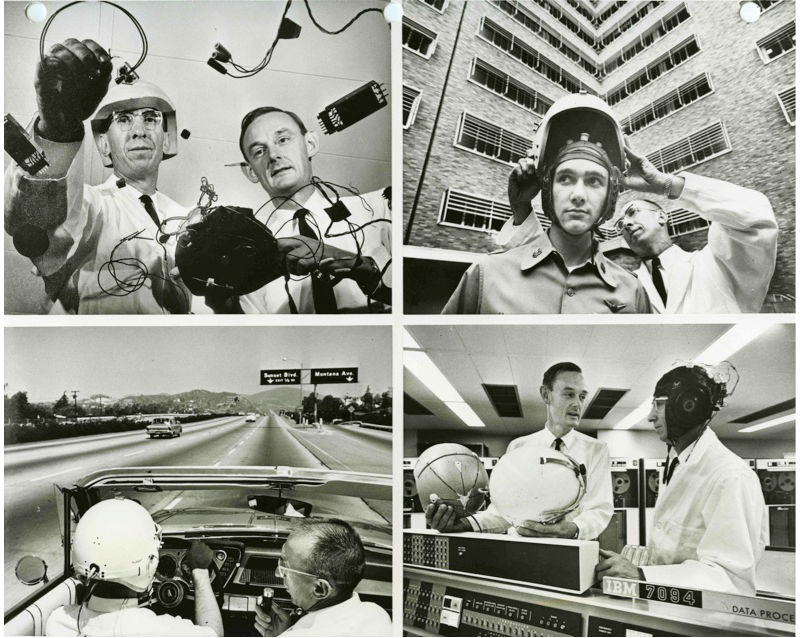This is a composite image consisting of four vintage black-and-white photographs, likely from the 1950s or earlier, detailing a scientific experiment involving two men who could be scientists. The top-left photo shows the two men amidst floating technical equipment, suggesting a zero-gravity environment, with one man wearing safety goggles and a helmet, and the other in a white shirt and tie. The top-right image captures one man in a helmet, having it adjusted by the other man, in front of a tall building. The bottom-left photograph depicts the helmeted man driving an old-style vehicle, possibly on Sunset Boulevard, while the other man, appearing to conduct an interview, is seated beside him, holding a microphone. Finally, the bottom-right image shows the two men in a laboratory crowded with vintage electrical equipment, with one man holding the helmet, exemplifying the era's experimental ambiance.